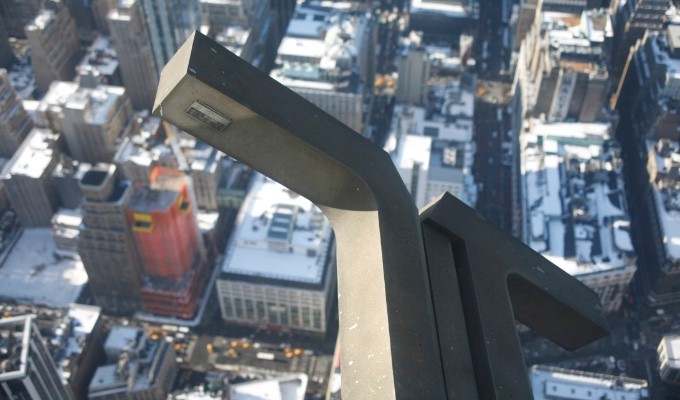An overhead view of a city captures a sprawling urban landscape below, rendered with some blurriness that obscures finer details. Numerous skyscrapers dominate the scene, with one prominently red building standing out among the mostly grey and white structures, which cast noticeable shadows. The rooftops of some buildings are outfitted with visible air conditioner equipment. The streets below are lined with numerous cars, contributing to the sense of bustling traffic. In the foreground, a strange, T-shaped metal beam or girder protrudes into the frame, angling from the upper left to the lower right. This metal object, gray with hints of brown and seemingly turned at right angles, adds an element of intrigue. The photograph, taken during a bright day with no visible clouds, features no identifiable landmarks, people, or animals, enhancing its ambiguous, almost surreal quality.